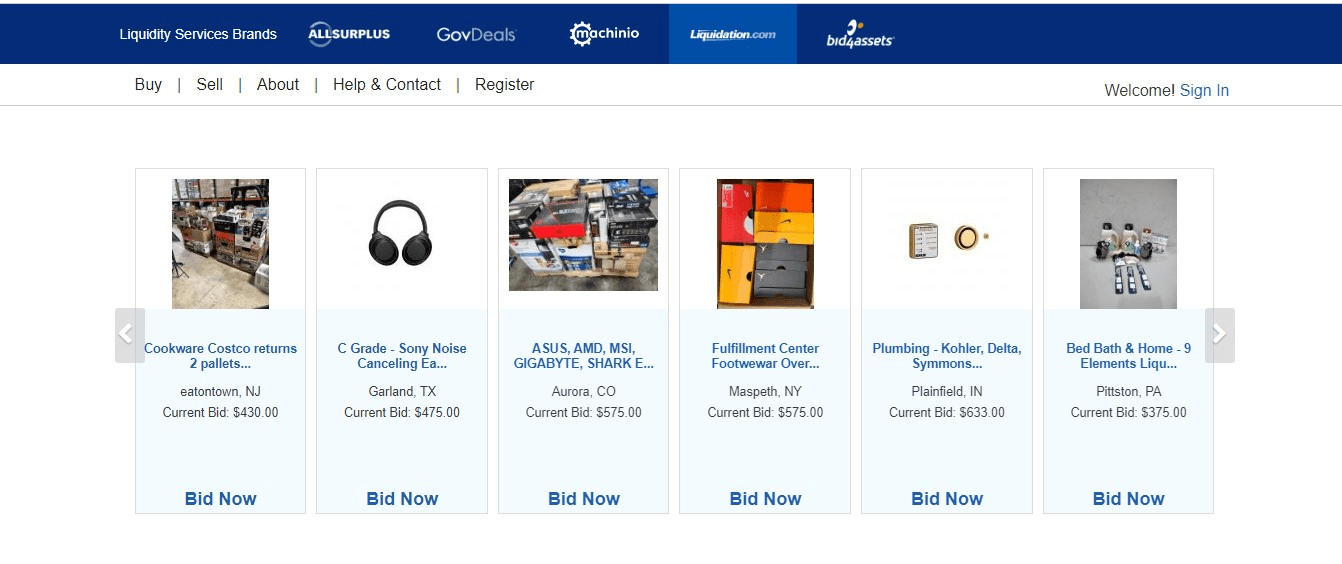The image depicts the homepage of the Liquidity Services Brands website, showcasing various brand names and sections. Prominently featured is the brand "AllSurplus," alongside icons for "GovDeals" and potentially "Bud Assets," though the text is somewhat unclear. These brands are listed in the upper blue banner of the page. Below this banner, navigational tabs are arranged from left to right: "Buy," "Sell," "About," "Help," "Contact," and "Register." On the far right, the banner warmly greets users with "Welcome!" followed by a "Sign In" option highlighted in blue.

Beneath this banner, a carousel of images displays various auction items. The first image is of cookware with the description "Costco returns two pallets," followed by a button labeled "Bid Now." The following image shows headphones labeled "C-Grade selling noise-canceling," with the location noted as Garland, Texas, and a current bid price of $475. Additional rotating images display items from brands such as ASUS, AMD, MSI, Gigabyte, and Shark, as well as categories like footwear, plumbing, bed and bath, and home goods. Each image includes relevant descriptions and a "Bid Now" button at the bottom.